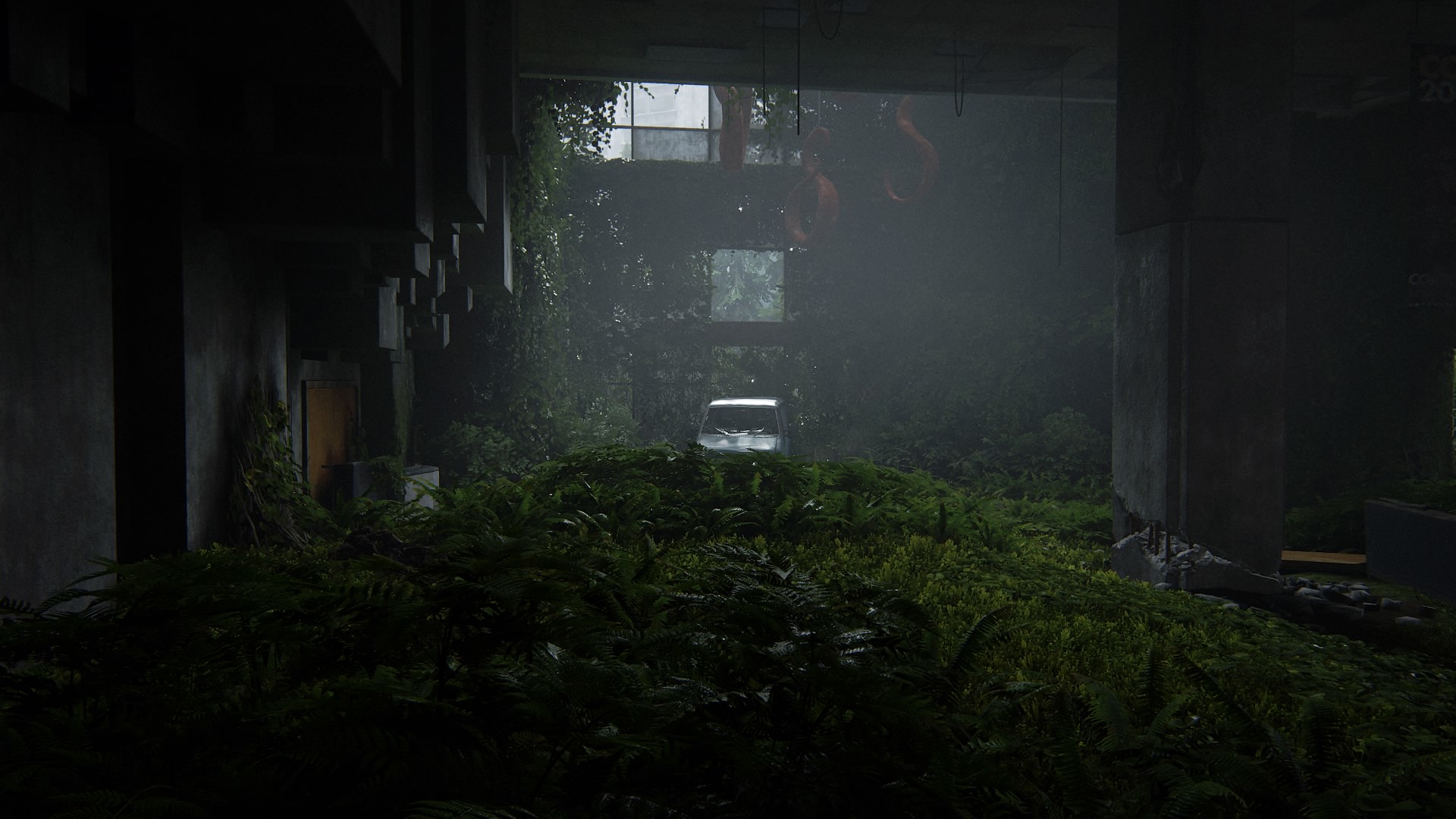This intriguing photograph appears to be taken in an underground setting. The walls are painted black, creating a stark contrast with the floor, which is overgrown with lush greenery and weeds, giving an unexpected juxtaposition of nature indoors. In the middle distance, there is a small, square-shaped, compact car. Suspended from the ceiling above the car are large, vibrant red hooks, adding an industrial element to the scene. To the upper left of the image, several window panes allow natural light to filter through, casting an ethereal glow across the space. The overall atmosphere is enveloped in a haze, contributing to a misty, somewhat surreal ambiance.